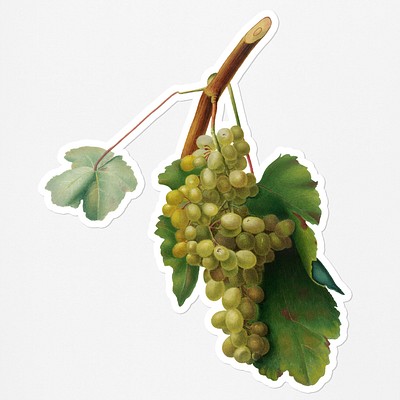This image is a highly detailed drawing or painting of a stalk of green grapes set against a solid light gray background. The main focus is a large bundle of green grapes, appearing juicy and varying in shades due to the way light interacts with their surfaces. They are clustered densely, possibly totaling around 50 grapes. The grapes hang directly from a brown stem, which extends from the middle of the composition and sprouts a few thin twigs and green leaves. One prominent, lighter green leaf is attached toward the center-left, while darker green leaves are positioned toward the bottom and right. A delicate white outline traces the contour of the brown stem, the twigs, and the grapes, enhancing the clarity and precision of the artwork. The overall image suggests a high level of craftsmanship, likely done with a green pencil or paint, emphasizing the natural richness and texture of the fruit and foliage.